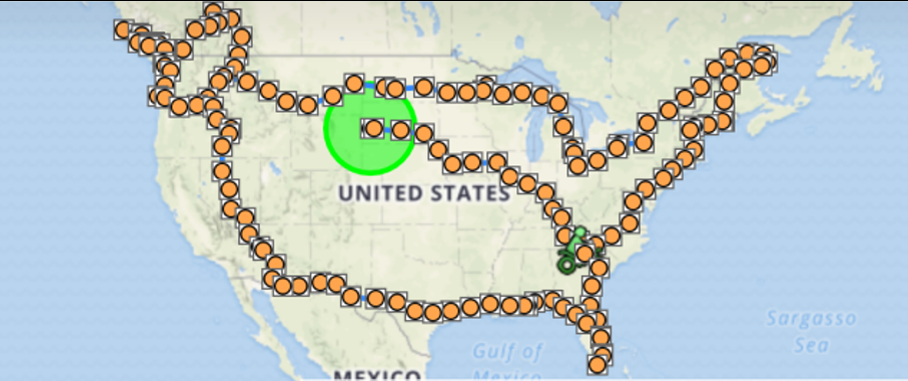The image is a detailed map of the United States, which includes parts of Canada at the top and Mexico at the bottom. The map features a pixelated blue background representing the water bodies, with labels for the Sargasso Sea and the Gulf of Mexico in darker blue. The United States is drawn in beige with olive green areas denoting the mountains.

A prominent lime green circle, outlined by a darker lime green ring, is positioned just to the left of the Midwest, above the words "United States" in bold, black uppercase letters. This circle appears to be a starting point for a highlighted route. This route is marked by several orange circles outlined in black and surrounded by gray squares. These orange circles form a path that begins in the upper Midwest, travels down, and circles through various regions.

The route traces down to the Georgia area, moves across the southern states like Texas and Louisiana, passes through the Gulf Coast down to Florida, and then moves up the East Coast. It extends across the top of the United States, dipping into parts of Canada, before sweeping back through the western states such as Washington, Oregon, and California. The path loops back to the initial lime green circle in the upper Midwest.

Additionally, the map features a lime green silhouette of a man on a bicycle, with the bicycle itself depicted in dark green, located around the Georgia area, suggesting a journey or a trip undertaken across these regions.